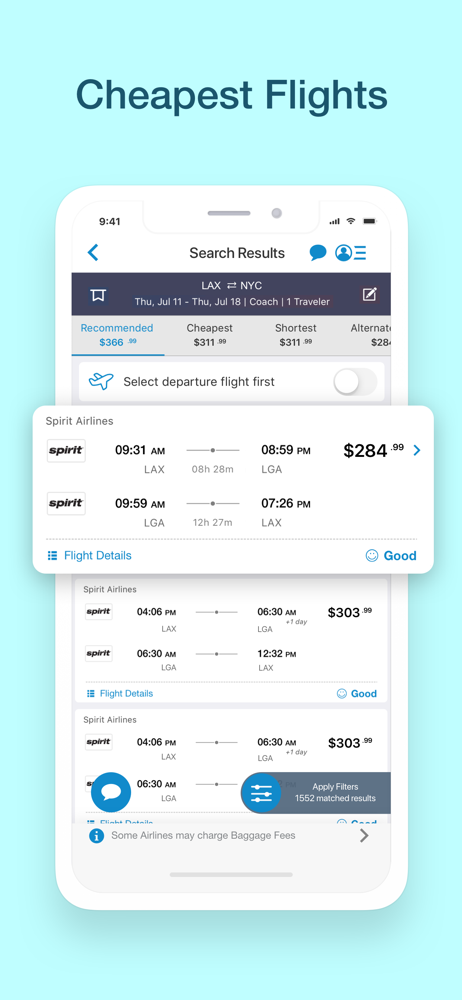Here is the cleaned-up and detailed caption:

---

This promotional image showcases a flight research and booking software interface against a light blue background. The banner reads "Cheapest Flights" in a darker blue font. Displayed is a smartphone screen with search results for flights from Los Angeles (LAX) to New York City (LGA), set for Thursday, July 11th through Thursday, July 18th. The search parameters include coach class and one traveler. The results are organized into columns labeled "Recommended," "Cheapest," "Shortest," and "Alternative."

Highlighted on the screen is a pop-up window for Spirit Airlines, featuring a flight priced at $284.99. Other flights in the results fall around $303.99. A toggle switch is available for selecting the departure flight first. Additionally, the interface notes that filters have been applied, showing a total of 1,532 matching results, and it also mentions that some airlines may charge baggage fees.